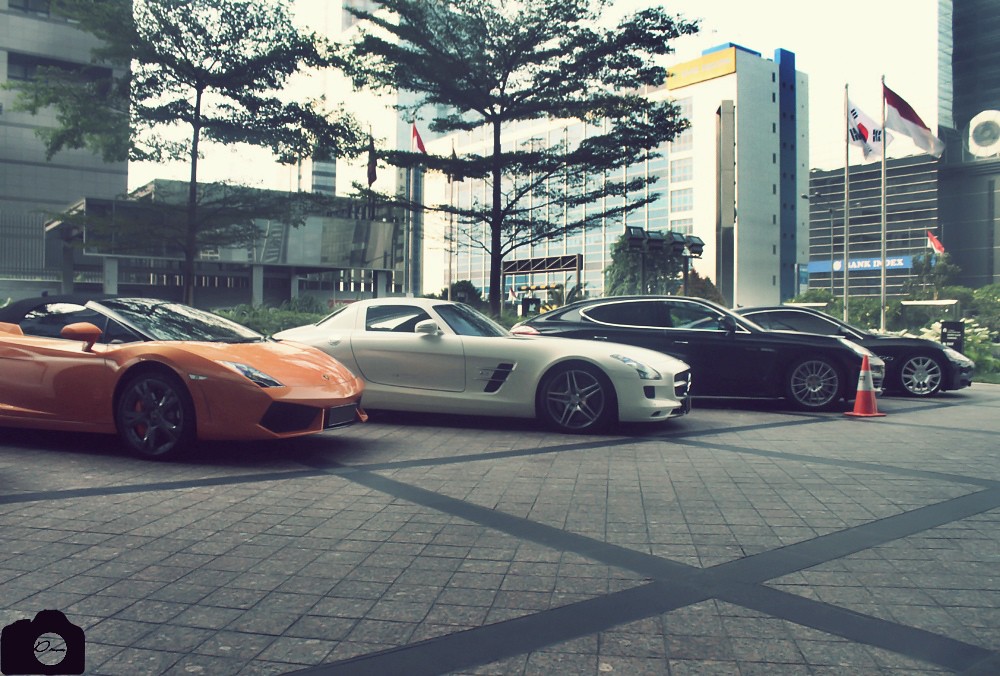This vibrant outdoor photograph captures a row of four high-end exotic cars parked diagonally on a stone-tiled parking lot. The lineup includes a striking orange convertible Lamborghini, followed by a sleek white two-seater, and two black luxury cars, one of which might be a Ferrari. The cars, with their shiny, expensive wheels, are faced towards the right. An orange and white caution cone stands prominently in the foreground. In the background, a large white building with yellow and blue trim can be seen, along with two flagpoles; one displaying the South Korean flag and an unidentified flag. The scene is set against a backdrop of several high-rise buildings, possibly suggesting a bustling cityscape such as Seoul, under a clear blue sky.